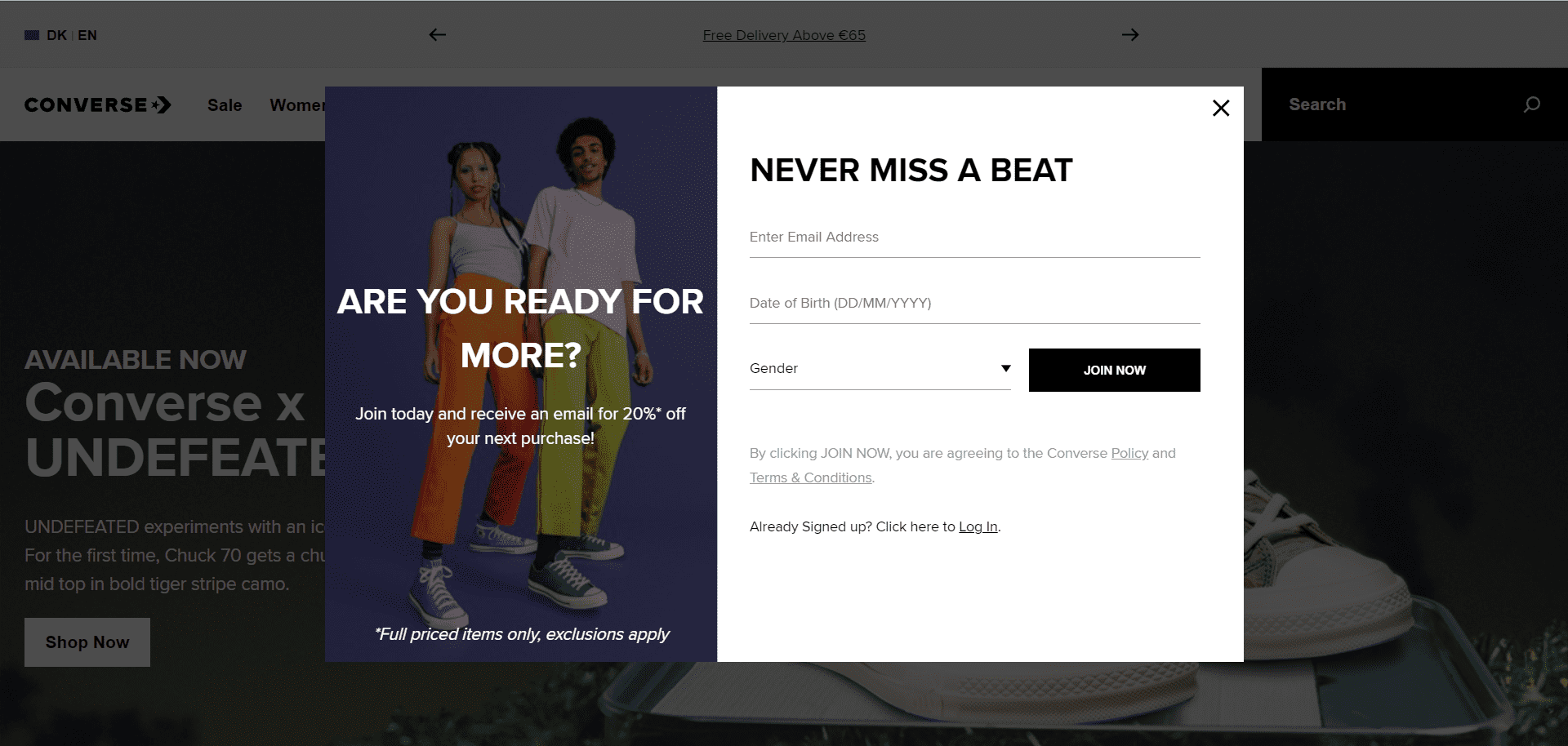The image depicts a pop-up dialogue box typically encountered upon visiting a website for the first time. At the top-right corner of the box, the text "Never miss a beat" appears in bold, drawing immediate attention. Below this bold heading is a text input field labeled "Enter email address," inviting users to provide their email information.

Following the email input field, there is a section for entering "Date of Birth," with a placeholder indicating the required format as (date/month/year). Adjacent to this, a dropdown menu is available for selecting the user's gender.

To the right of the gender selection menu, a prominent black button labeled "Join Now" encourages users to complete their information submission. The final line of the pop-up box contains a disclaimer in smaller text that reads, "By clicking Join Now, you're agreeing to the customer policy and terms and conditions," informing users about the consent required for proceeding.

The overall design of the dialogue box balances textual elements with input fields effectively, guiding the user smoothly through the subscription process.